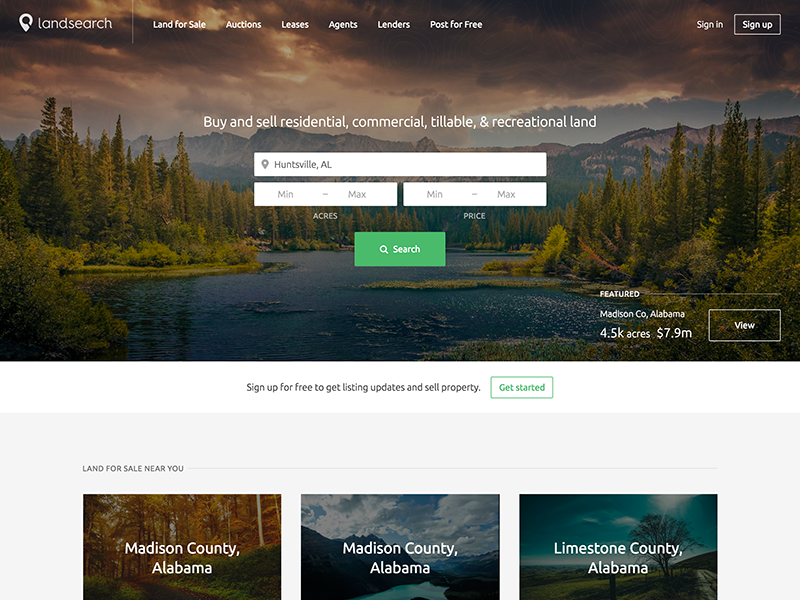The website's homepage features various elements designed to facilitate land searches and transactions. At the top, there is a navigation bar with options such as "Land Search," accompanied by a small search icon, "Lands for Sale," "Options," "Leases," "Agents," "Lenders," "Post for Free," and on the far right, buttons for "Sign In" or "Sign Up."

In the central section, a banner highlights the website's purpose with the text: "Buy and Sell Residential, Commercial, Tillable, and Recreational Land." Below this, a picturesque image is displayed, showcasing a dramatic cloudy sky with layers of gray clouds intermingled with orange and yellow hues. The backdrop features distant mountains and a dense array of evergreen trees on both the left and right sides. In the foreground, a tranquil lake mirrors the scenic vista. Superimposed on this image is a white banner that reads "Huntsville, Alabama," accompanied by a gray location marker icon.

Below the main image are interactive search filters: two banners, one for "Minimum to Maximum Acres" and the other for "Minimum to Maximum Price," followed by a prominent green search button labeled "Search."

On the right side of this section, a "Featured" label in white introduces a prominent listing: "Madison County, Alabama, 4.5 thousand acres, $7.9 million." Beneath this, a white call-to-action box encourages users to engage further. It includes options to "Sign Up for free to get listing updates and sell property." Next to this box, a green banner with the text "Get Started" invites immediate action, and below it is a prompt about planning for sale periods.

At the bottom, three thumbnail images provide a visual preview of properties available in Madison County, Alabama. The first thumbnail shows a vibrant forest with autumnal colors of red and yellow. The middle image captures a clear blue sky with expansive clouds, mountains, and a lake, emphasizing the region's natural beauty. The last image focuses on Limestone County, Alabama, showcasing a sprawling sky with clouds and undulating mountainous terrain.